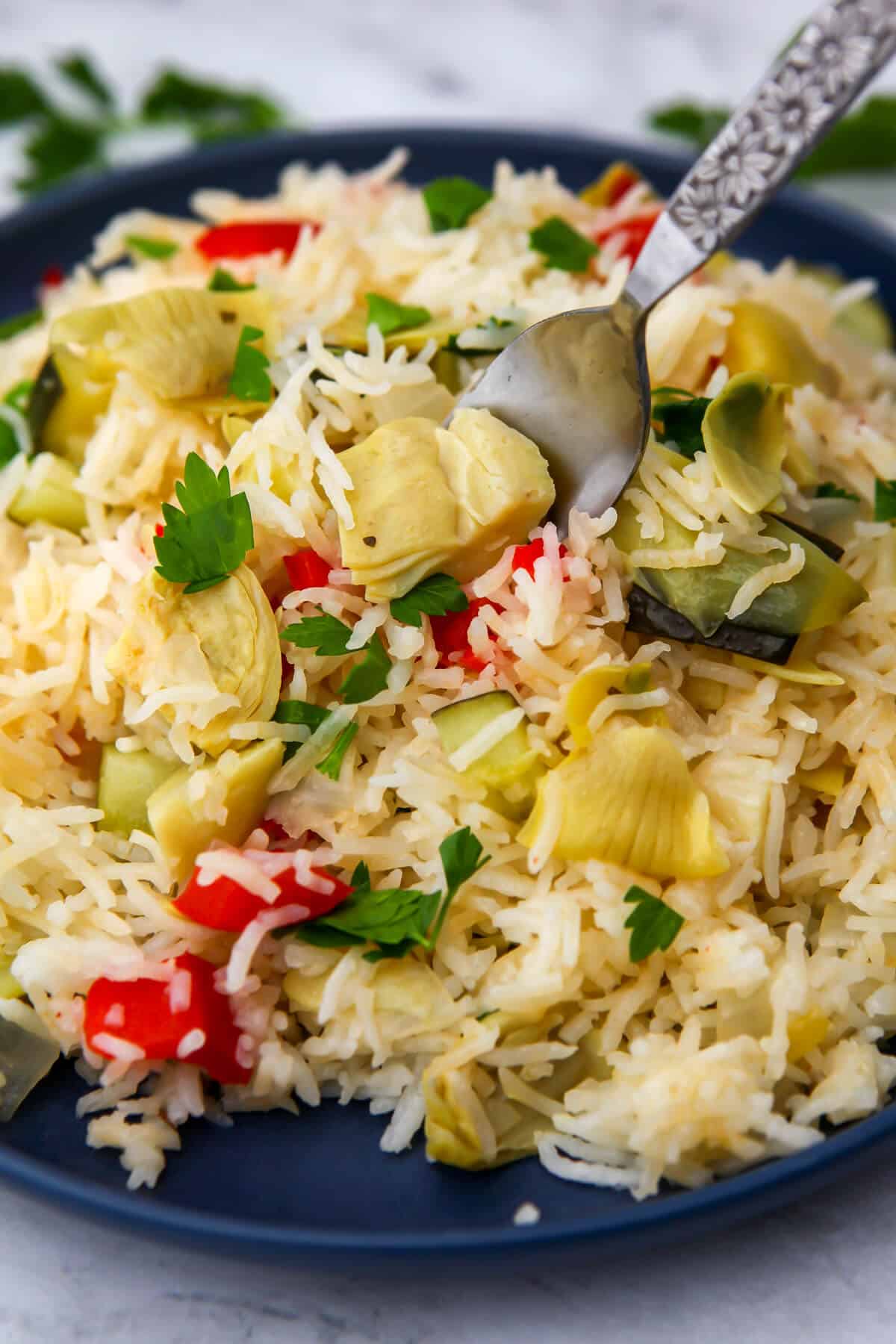The image showcases a vibrant culinary arrangement on a navy blue plate with an upward-curved lip, set on a light gray marble table. The plate is densely covered with moist white rice, topped with a colorful medley of ingredients. Scattered throughout the dish are fresh green leafy vegetables, likely basil or parsley, adding a touch of freshness. Bright red slices of either peppers or tomatoes provide a striking contrast. Yellow artichoke hearts, with their layered appearance, bring a rich texture to the composition. A silver spoon with an intricate sunflower design on the handle is poised on the upper right corner, ready to scoop up a portion of the delightful dish. This meticulously arranged and visually appealing plate captures the essence of a well-crafted, flavorful meal.